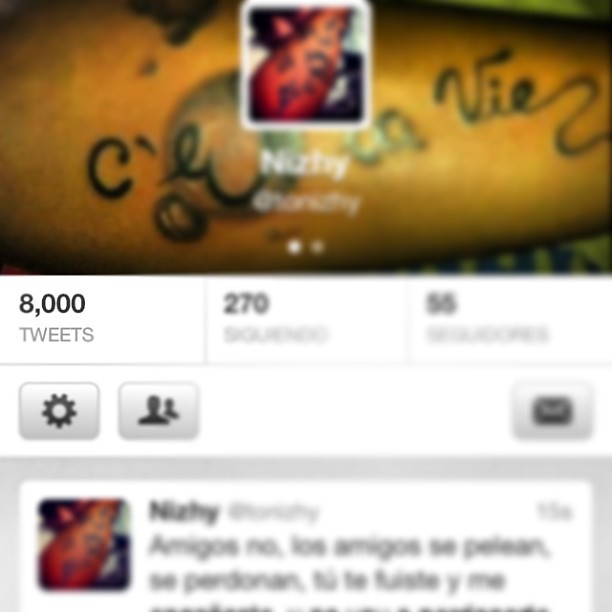This image is a heavily blurred close-up screenshot of a Twitter account displayed on a phone. Prominently, it marks the user's 8,000th tweet, clearly visible amidst the blur. The header features a script suggesting "C'est la vie," likely a tattoo on someone's forearm, adding a personal touch. An inset of a red and black logo overlays part of this background. Although most of the text is indecipherable, there are fragmented mentions of followers—270 in number—and following 55 accounts. The account seems to belong to someone possibly named Nitzy or NIZHY. Alongside the account stats, there are standard icons, such as the gear for settings, and friend and mail icons. A post below, potentially in Spanish, contains phrases like “amigos, no los amigos,” though it's largely unreadable. The details emphasize the effort to celebrate a social media milestone amidst a blend of visual elements and multiple languages.